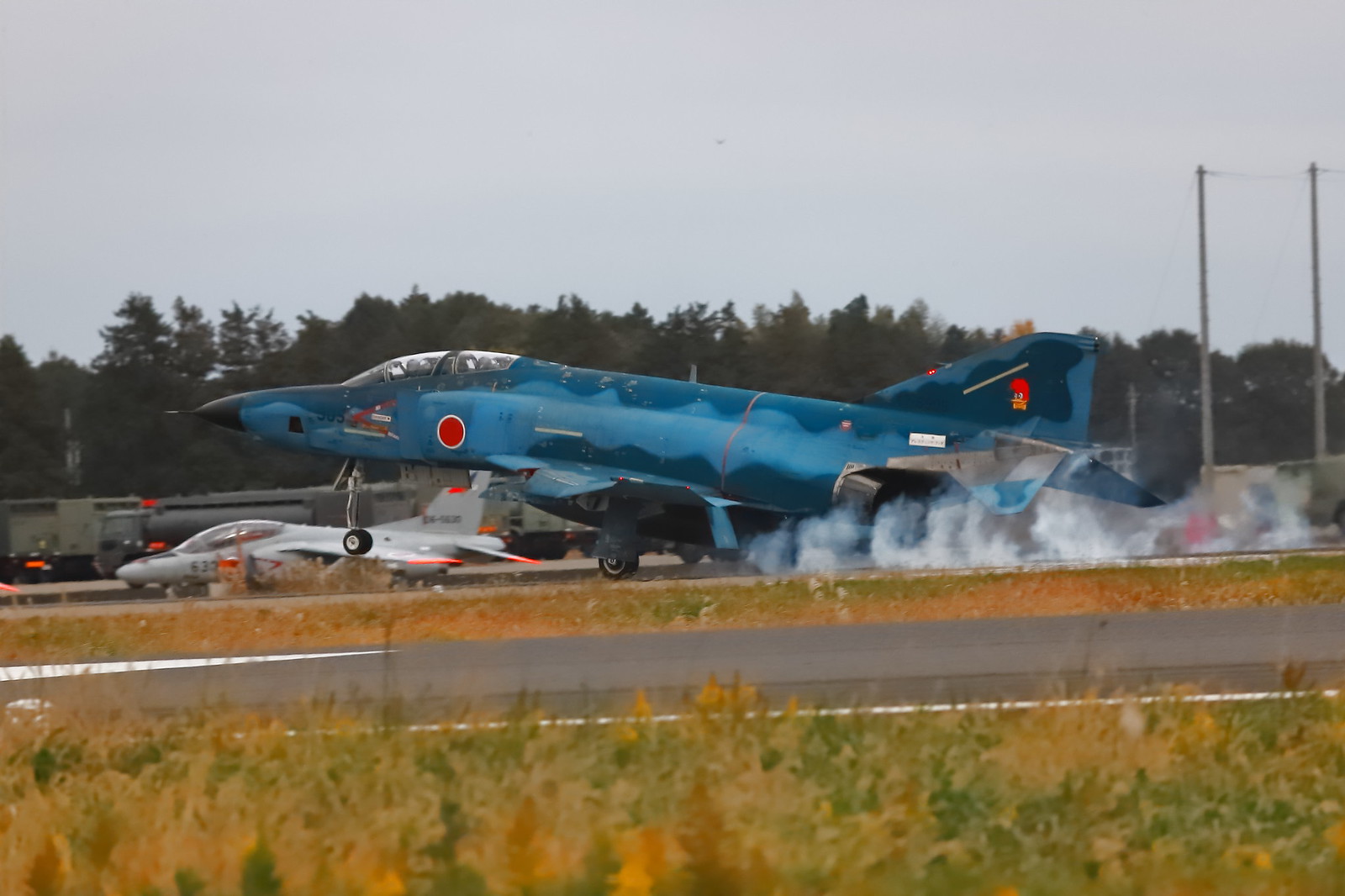The image is a detailed color photograph of two small planes on a runway, set against a dreary, overcast sky. In the foreground, a strip of grass borders the cement runway. The main plane in focus is a blue jet with a distinctive design featuring scalloped blue waves and a darker blue section on either side of a red dot located beneath the cockpit window. Woody Woodpecker is illustrated on its tail, which angles upwards. The jet is in the process of taking off; the nose is lifted, and the front landing gear is off the ground. Plumes of white smoke emerge from the rear wheels as they skid along the runway. Following this aircraft, another smaller, silver plane with red wingtips is stationary on the tarmac. The scene also includes two electrical poles in the background and a backdrop of trees, adding depth to the composition.